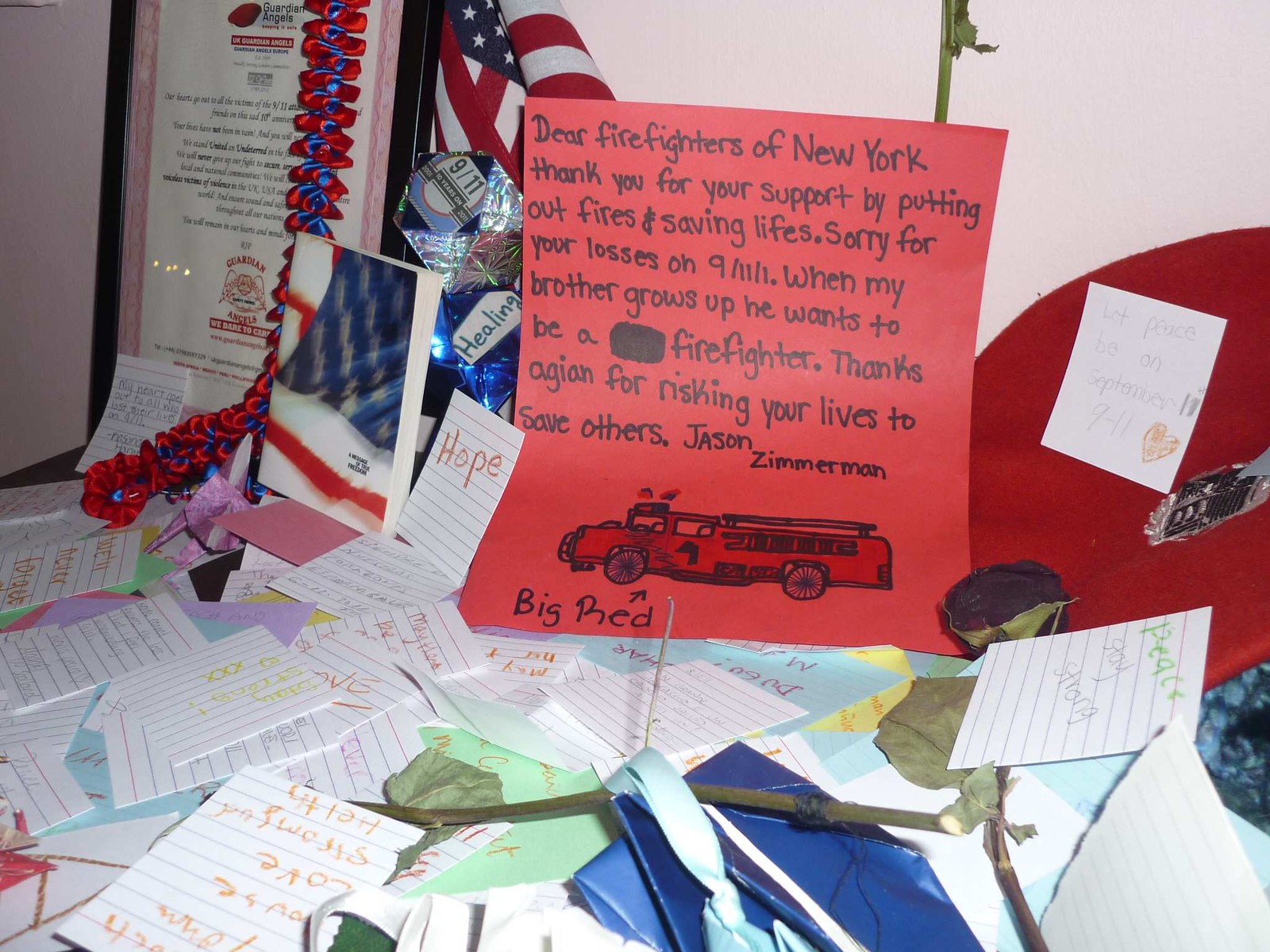The image depicts an indoor display featuring an assortment of scattered handwritten notes and greeting cards, primarily from children. These notes are written in various markers and crayons on items such as index cards, ruled notebook paper, and colored construction paper. Prominent messages include words like "hope," "peace," "love," "we'll never forget," and references to "September 11."

Among the display, a large red card stands out with a heartfelt message addressed to the "Firefighters of New York," expressing gratitude for their bravery and condolences for the losses experienced on September 11, 2001. The card, authored by Jason Zimmerman, includes a drawing of a firetruck labeled "Big Red" and mentions the aspirations of his brother to become a firefighter.

In addition to the notes, the scene includes a small American flag, designer ribbons in red and blue, and a dead rose plant placed on a table. Notably, there is a black-framed certificate of appreciation with text referencing "guardian angels," expressing solidarity and remembrance for the 9/11 victims. The certificate reflects messages of unity and the continued fight for securing local and global communities.

Overall, the image portrays a touching tribute filled with personal notes and mementos, commemorating the heroism and sacrifice of firefighters and victims from the tragic events of September 11.